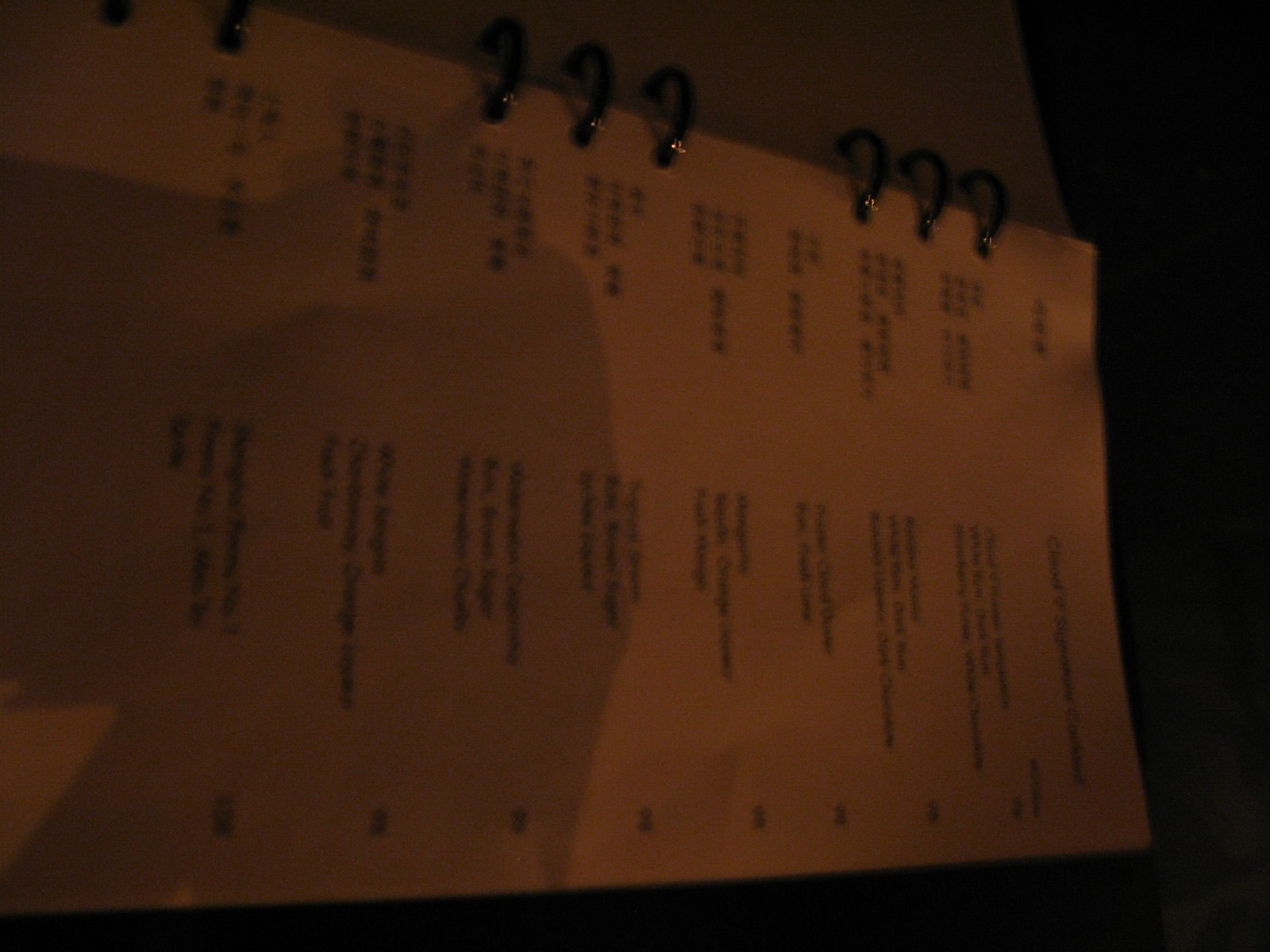In the image, the background is predominantly dark, with a strong shadow enveloping the left side and obscuring half of a piece of white paper, which appears to be part of a notebook. The notebook's binder rings are clearly visible, with three black rings centralized in the upper portion of the image and another set of three rings located approximately three inches to the right. The white paper, taking on a slightly dark yellow hue due to the dim lighting, has areas of text that remain mostly indistinct and blurry. In the upper left corner, a small section of text is barely visible, with the word "chapter" more discernible about three inches to the right. The lower right portion of the image likely contains page numbers, albeit blurry and unclear due to the overall shadowy and dark context.